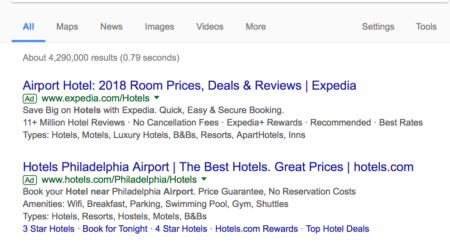This rectangular image, oriented horizontally with its longer side extending from left to right, appears to be a screenshot of a search engine result, likely from Google. The top section features a grayish border containing navigational options, including "All," "Maps," "News," "Images," "Videos," "More," and on the far right, "Settings" and "Tools." Evidently, the "All" tab is selected, as indicated by its blue underline, while the other options are displayed in gray text.

Immediately below this border, the search results summary indicates there are approximately 4,290,000 results retrieved in 0.79 seconds. The first result prominently displays the title "Airport Hotel 2018 Room Prices, Deals, and Reviews from Expedia" in dark blue text. Just beneath this, the link is highlighted in green text, formatted as "ad www.expedia.com/hotels."

The accompanying description in black text promotes Expedia's offerings: "Save big on hotels with Expedia—quick, easy, and secure booking. 11+ million hotel reviews, no cancellation fees, Expedia Plus rewards." It also lists various types of accommodations available through Expedia: "Recommended, Best Rates. Types: Hotels, Motels, Luxury Hotels, B&Bs, Resorts, Apartment Hotels, Inns."